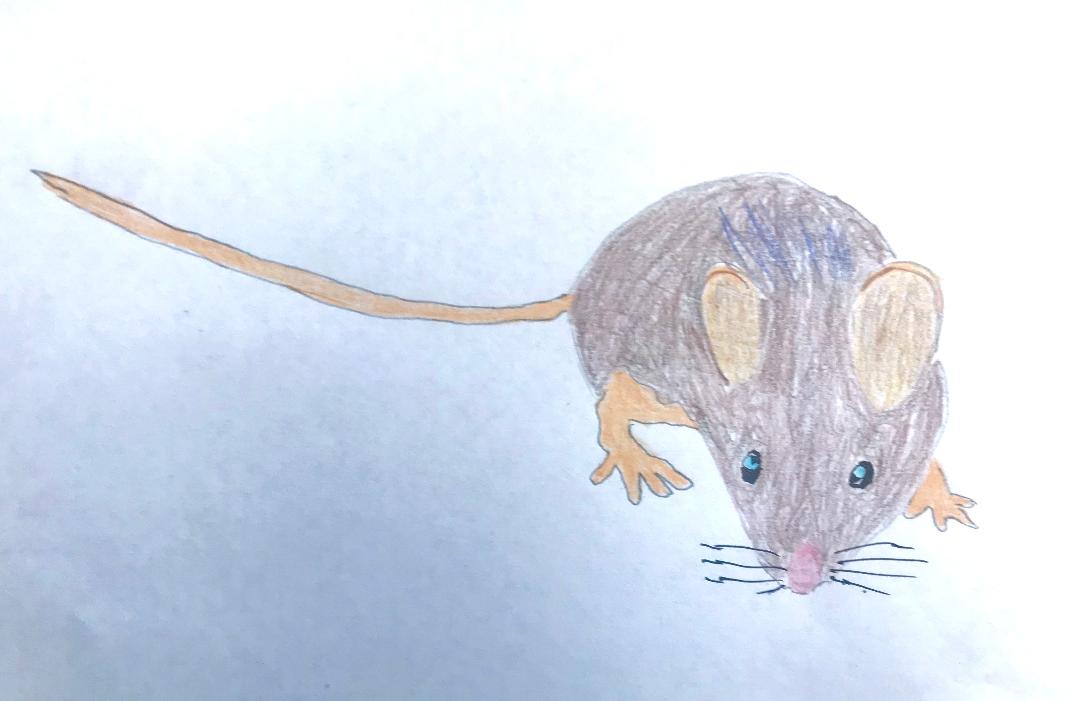This image depicts a detailed colored pencil and crayon drawing of a mouse, possibly a rat, on a white piece of paper with slight shadows. The rodent is positioned facing the viewer, with a grayish body accented by blue on its back, covered in fur with visible longer hairs. Its large, tan ears and pink nose stand out prominently, and it has eight black whiskers, four on each side. The mouse's tail, also tan, extends to the left. It has a pair of tan legs visible, one on the left and one on the right. The eyes are a dark blue with aqua blue pupils, enhancing the creature’s lifelike appearance. The drawing, although detailed, shows distinct colored pencil strokes, indicative of being created by a young artist, likely in elementary school.